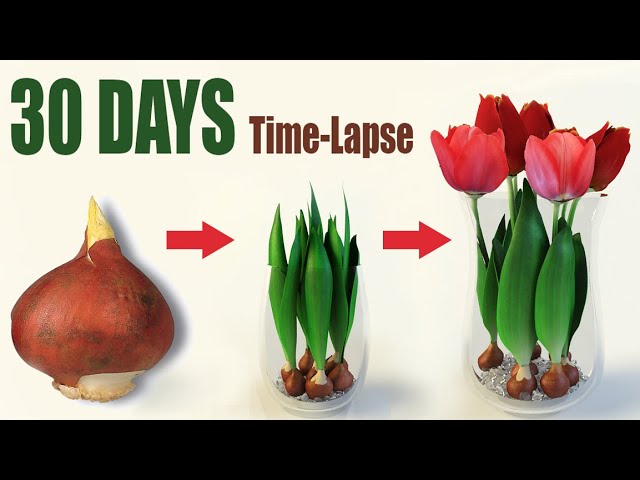This detailed image illustrates the 30-day time-lapse growth cycle of a tulip bulb, accompanied by clear visual guides and annotations. Set against a white background framed by a one-inch black border at the top and bottom, the sequence begins on the left with an image of a reddish-brown tulip bulb with white and tan accents. The large green text "30 days" and the phrase "time-lapse" in dark reddish brown are prominently displayed at the top.

An arrow points to the central stage, where the bulb has been placed in a glass container. Here, the bulb has sprouted green leaves that extend beyond the jar's rim. This secondary phase shows either five or seven bulbs beginning to grow. Another red arrow leads to the final stage on the right, where the fully matured tulips are in full bloom with vibrant red flowers and lush green stems and leaves, still housed within the same glass container. The image effectively captures the transformation from bulb to blooming flower, beautifully illustrating the life cycle of a tulip.